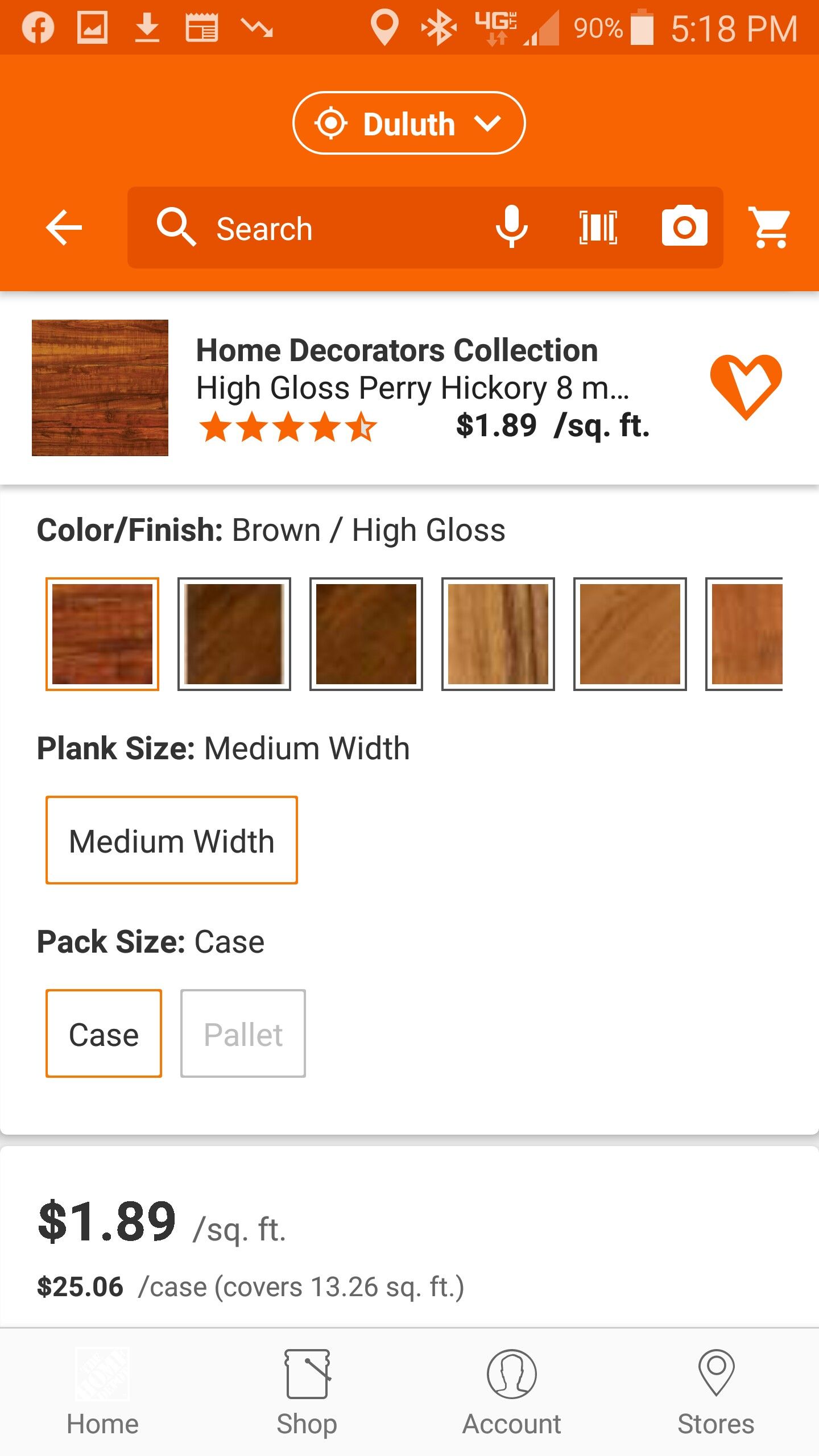Screenshot from a Mobile Device

At the top left corner are several icons in sequence: a Facebook icon, a picture icon, a download icon, an article icon, a market icon indicated by an arrow, a location icon, a Bluetooth icon, the 4G symbol, and a signal bar showing two bars of signal strength. Beside these is a battery icon displaying 90% and the time noted as 5:18.

Below the status bar, there's an oval button labeled "Dulles" accompanied by a drop-down arrow. Adjacent to it is a rectangular search box featuring three embedded icons and an external shopping cart icon. On the left side of the screen, there's a back arrow housed within an orange banner.

The main section of the screen is dedicated to a product listing under the title "Home Decorators Collection." This listing includes a featured image of wooden flooring with customer ratings displayed beneath. To the right of the ratings is a heart icon.

The product details begin with the text "Color / Finish" in bold, specifying "Brown / High Gloss" followed by corresponding thumbnail images of different colors and finishes of the flooring. Below this, "Plank Size" is listed as "Medium Width" with an accompanying button. The next detail notes "Pack Size" with "Case" highlighted.

The pricing is clearly indicated as "$1.89 / square foot" and "$25.06 / case" with various actionable icons situated at the bottom of the screen.